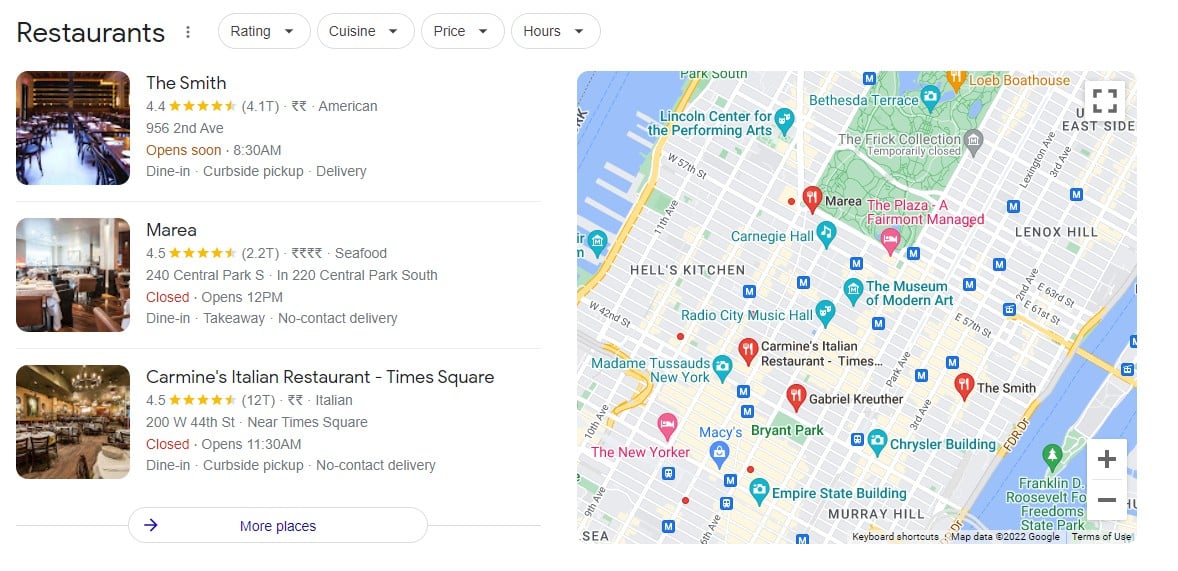The image depicts an interactive map interface of a dining guide application. At the top left corner, there is a "restaurant" tab, which is accompanied by three vertical dots. Next to this, there are additional filter options including "rating" with a down arrow, a pill-shaped icon likely indicating a filter, another pill-shaped icon labeled "cuisines" with a down arrow, followed by a "price" filter also with a down arrow, and an "hours" filter with the same down arrow.

In the main section of the map interface, listings for several restaurants are displayed: The Smith, Maria, and Carmine, an Italian restaurant located in Times Square. These listings feature images of restaurant interiors showcasing dining halls filled with tables and chairs under various types of lighting.

On the right side of the image, there is a map illustrating the locations of food establishments within the vicinity, bordered by water on the top left and bottom right. The map includes functionality buttons such as zoom in/out (+/-), a full-screen mode, and colored icons in blue, red, and pink indicating different points of interest.

Each restaurant listing provides ratings, with Maria and the Italian restaurant both receiving 4.5 stars, while The Smith has a rating of 4.4 stars. At the bottom of the interface, there is a "more places" option accompanied by a right-facing arrow, suggesting additional listings can be viewed.